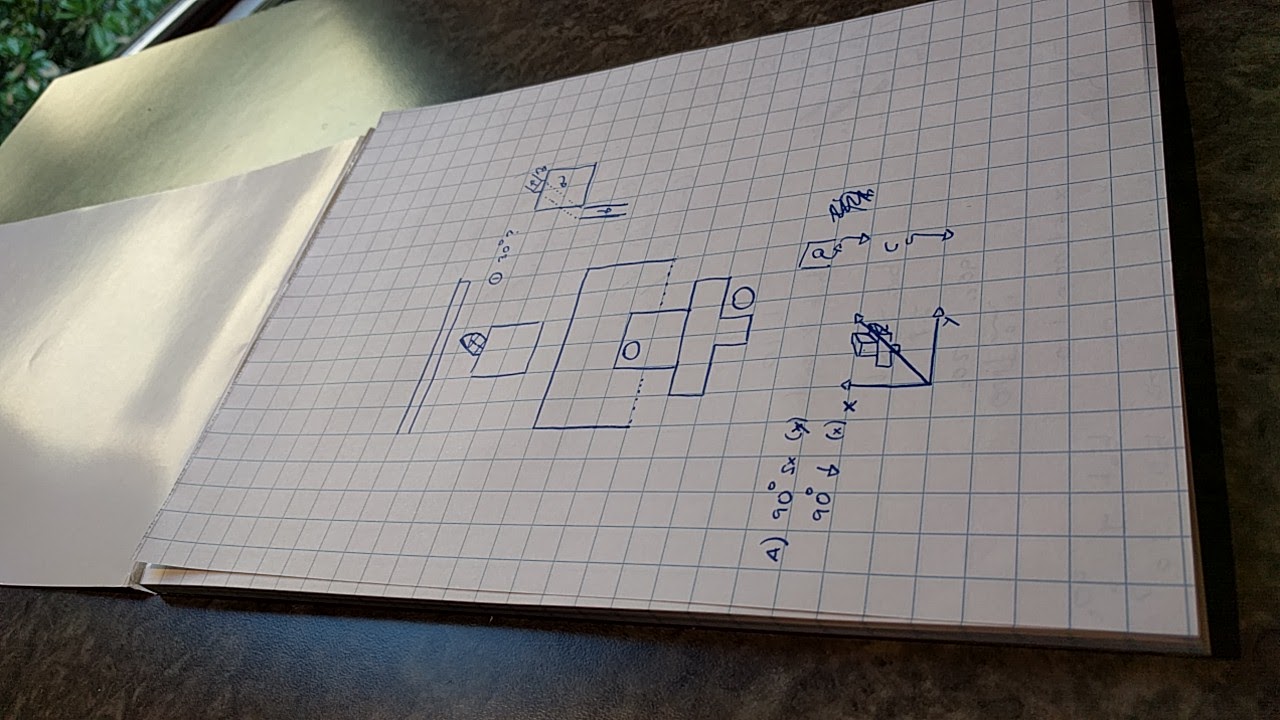The image presents an aerial view of an open notebook, positioned vertically and slightly tilted. The notebook features white pages with a blue square grid pattern, indicating it is designed for mathematical notation. The page on the right contains various equations, numbers, and shapes, possibly representing a student's schoolwork. The opposite page is blank, with light reflecting off its surface as well as the marble table on which the notebook rests. In the top left corner of the image, part of a plant, possibly a small tree, is visible, adding a touch of greenery to the scene. The overall composition highlights the reflective quality of the surfaces and the structured layout of the notebook's grid paper.